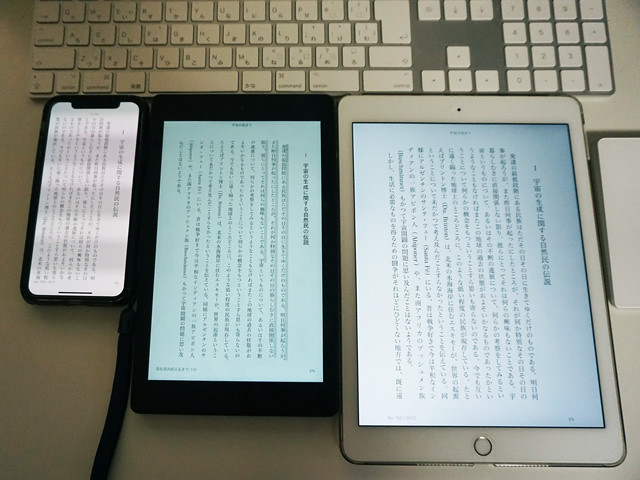The image depicts a collection of smart devices arranged on a flat white surface, likely a table or desk, in an interior setting illuminated by artificial lighting. The lighting creates noticeable shadows, making the left side of the image darker than the right. Positioned at the top of the image is a sleek, flat, silver keyboard with white keys and black lettering, resembling an Apple keyboard. Below the keyboard, three smart devices are aligned side by side, each displaying the same page filled with Asian characters, likely Chinese, running from top to bottom. On the left is a small, flat-screen smartphone; in the center is a medium-sized black tablet; and on the right is a larger, white tablet, possibly an iPad. The setup appears to be a well-organized, tech-centric workspace, capturing a moment of digital engagement in an indoor environment.